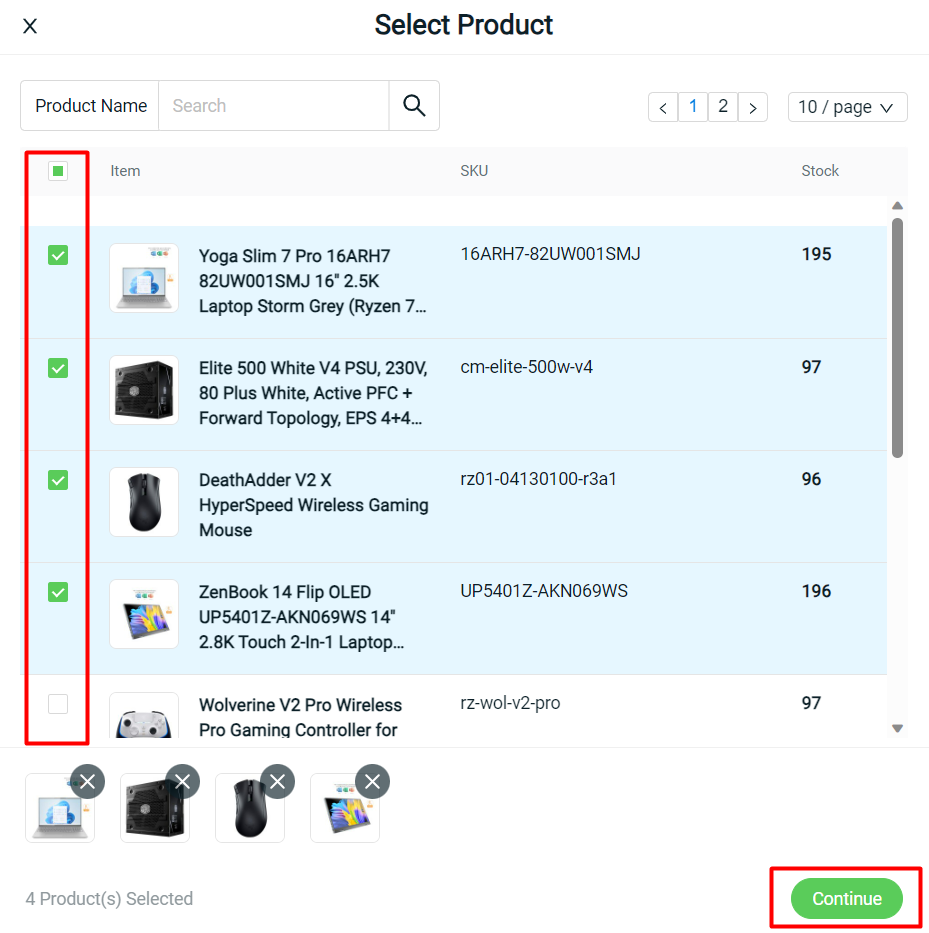Displayed in the image is a product selection and inventory page highlighting specifically chosen items. The selected products are highlighted in blue and include a Yoga Slim 7 Pro laptop, an Elite 500 white top, a Hyperspeed wireless gaming mouse, and a two-in-one laptop. Additionally, an unselected item—a pro wireless gaming controller—is also visible. Despite the presence of the controller at the bottom of the page, it appears to not be part of the currently highlighted selection. This page does not seem to be structured for direct product comparison, as the assortment includes diverse types of products. The layout and design of the page suggest it may be a unique inventory or selection interface rather than a typical order page.